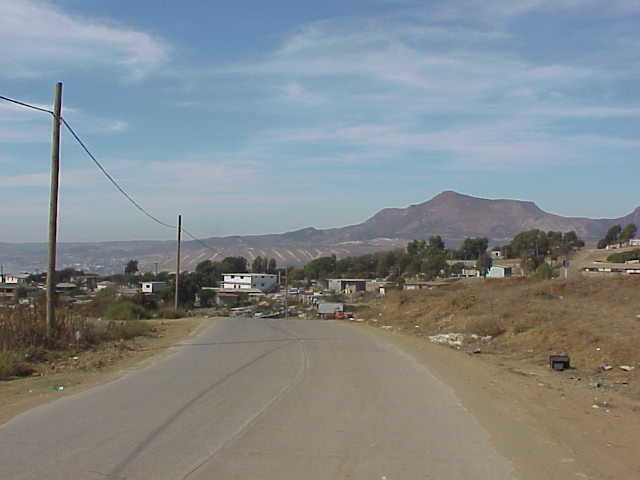A photograph depicts a desolate, rural road flanked by brown, dirt-laden fields on both sides. The road, which appears dirty and scattered with trash, is lined by a couple of electrical poles with wires stretching across the left side. In the distance, there are small, worn-down houses or buildings, hinting at a modest or impoverished area. Beyond these structures, there is a stretch of farming land or a possible vineyard, leading up to a looming mountain range that frames the horizon. The sky is filled with blue and white floating clouds, providing a sharp contrast to the brown and grey tones dominating the landscape. Overall, the scene evokes a sense of abandonment and bleakness, underscored by the unkempt surroundings and minimal vegetation.